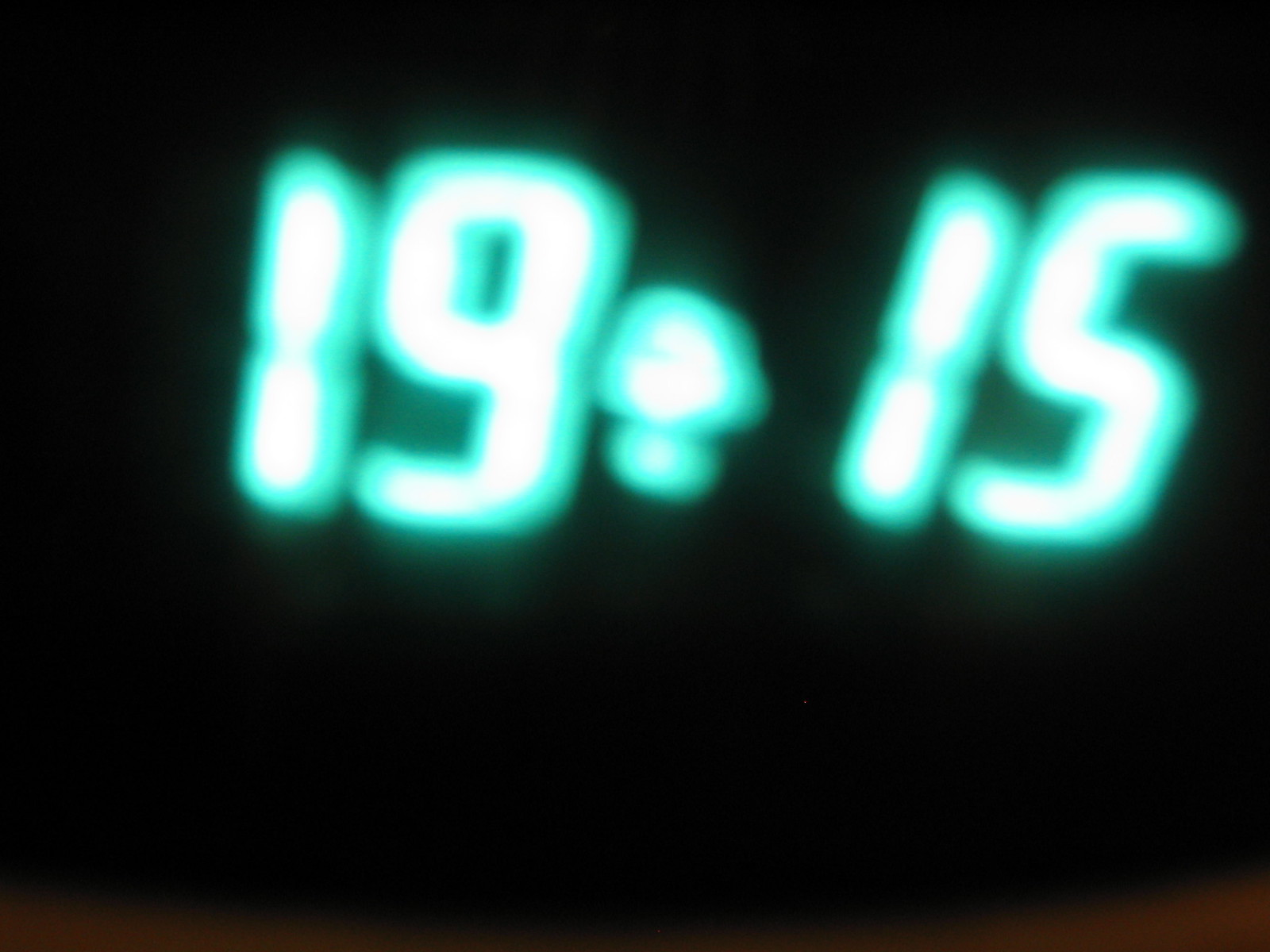A close-up photograph of a digital clock face dominates the frame. The black display is the sole focus, with neon green digits vaguely displaying the time, "19:15," equivalent to 7:15 PM in a 12-hour format. Due to the extreme proximity, the image is heavily out of focus, rendering the numbers blurred and slightly oversized. The details are so distorted that discerning the exact time requires focus, adding a layer of abstraction to the otherwise mundane moment captured.